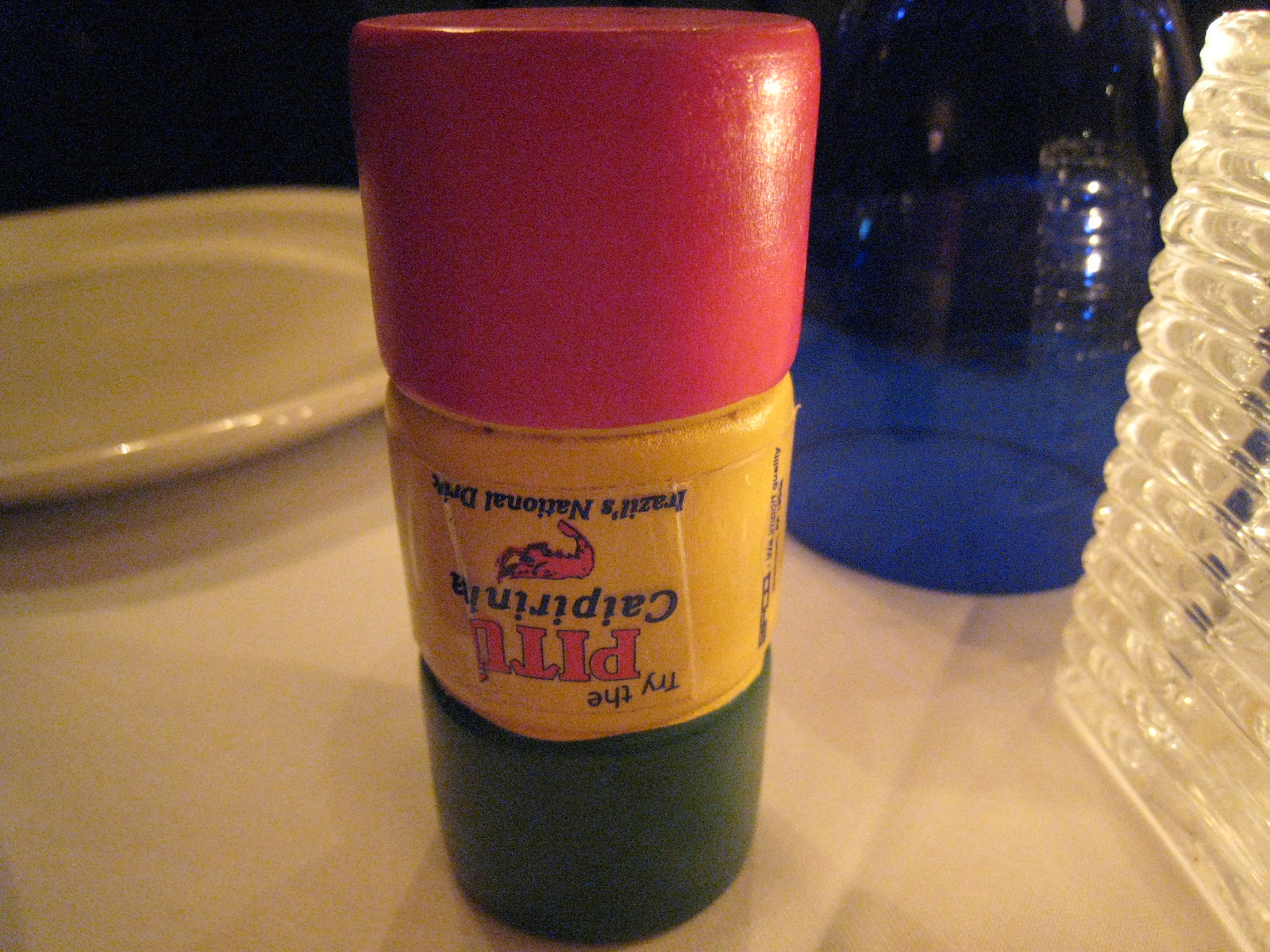The photograph captures a tabletop scene with a white tablecloth in a dimly lit room. Central to the image is an upside-down cylindrical tube featuring a green band at the bottom (actually the top), a yellow-white middle band, and a red band at the top (actually the bottom). The yellow-white middle band bears a crinkled label that is partially unreadable, though it contains text in black and red saying "Try the P2" or "Try the Pidou" and mentions "Brazil's National Drink." Additionally, there is an illustration of what looks like a shrimp or lobster on the yellow band. 

In the background, to the left sits a white ceramic plate, glossy under the lighting but empty, while to the upper right, an upside-down blue wine glass stands. On the lower right edge of the frame, there appears a clear, ridged, possibly square-shaped vase or container. This clear object features various ridges encircling it, which could also correspond with small round tubes. The overall setting is a table setup with decorative items.